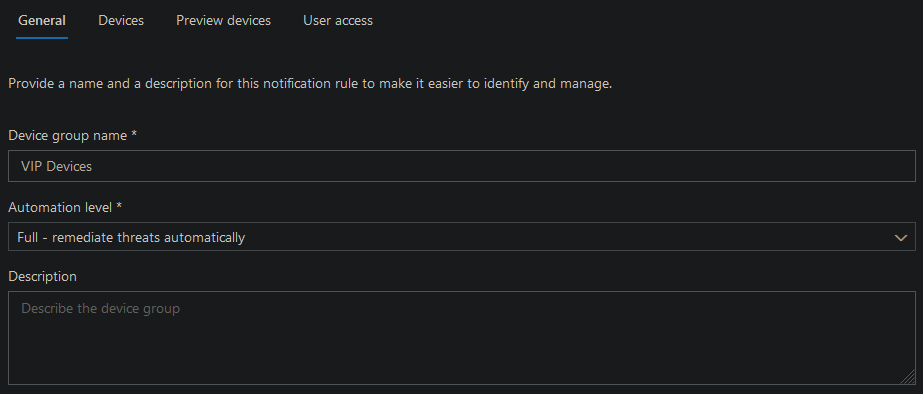The image displays a user interface with a completely black background. At the top left, several white tabs are visible, with the first tab, labeled "General" in bold and underlined in blue, indicating it is the currently selected tab. The subsequent tabs are "Devices," "Preview Devices," "User Access," each beginning with a capital letter but with normal font weight.

Below these tabs, a text prompt reads, "Provide a name and description for this notification rule to make it easier to identify and manage." Further down, in white text, the label "Device Group Name" appears next to an asterisk, indicating a required field. Adjacent to this label is a black rectangle with a white border, inside which the text "VIP" is written in all capital letters.

Next, the interface presents the label "Automation Level" marked with an asterisk, signifying it as another required field. Beside this label is a similar rectangular box, black inside with a white border, containing the word "Forward" in white capital letters. Below this box, a white arrowhead pointing downwards suggests a dropdown feature. 

Following some additional black space, the label "Description" is seen. Adjacent to it is another black rectangle with a white border containing placeholder text that reads, "Describe the device group."

This detailed caption comprehensively describes the elements and layout of the user interface depicted in the image.